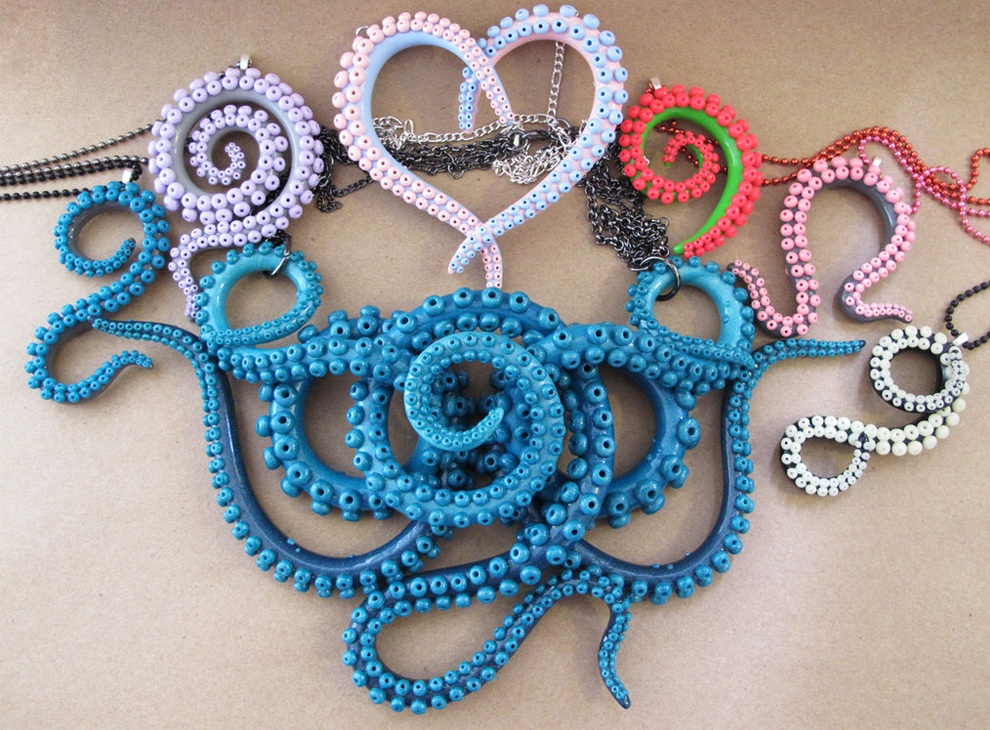The image showcases a vibrant and intricately designed collection of what appear to be jewelry pieces crafted to resemble octopus tentacles, likely made from plastic or rubber. The largest piece, a dark greenish-blue tentacle, is overlapped and stands out prominently in the center. Other pieces vary in color and form intricate shapes: a pale pink and blue tentacle forms a heart, while other tentacles are spiraled in hues of white, lavender, red, green, and a combination of pink and dark gray. Chains attached to several of these pieces suggest they may be wearable, possibly as necklaces. Displayed against a beige countertop, this elaborate arrangement highlights the creative fusion of marine-inspired art and jewelry.